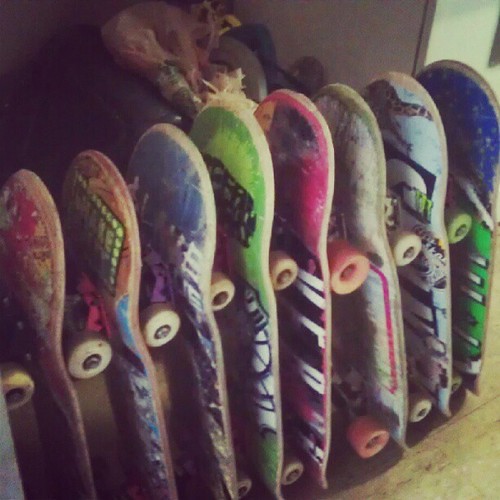This photograph captures a neatly arranged row of eight skateboards standing vertically on a wooden floor, their wheels aligned toward the left. Each skateboard is unique in color and design, contributing to an array of visual diversity. From left to right, the skateboards exhibit a variety of hues including red with a design, orange and blue with a yellow and black logo, predominantly blue with some white, lime green with black and white spray paint, red with white letters, green and white with a pink rectangle, light blue with black lettering, and a royal blue top with a lime green bottom featuring white and black large letters. The boards are standing wheel-to-board, packed closely together, and they form a slightly diagonal line from the bottom left to the upper right corner of the image. In the background, partially visible but indistinct items and the corner of a gray wall suggest a cluttered or artistic setting.